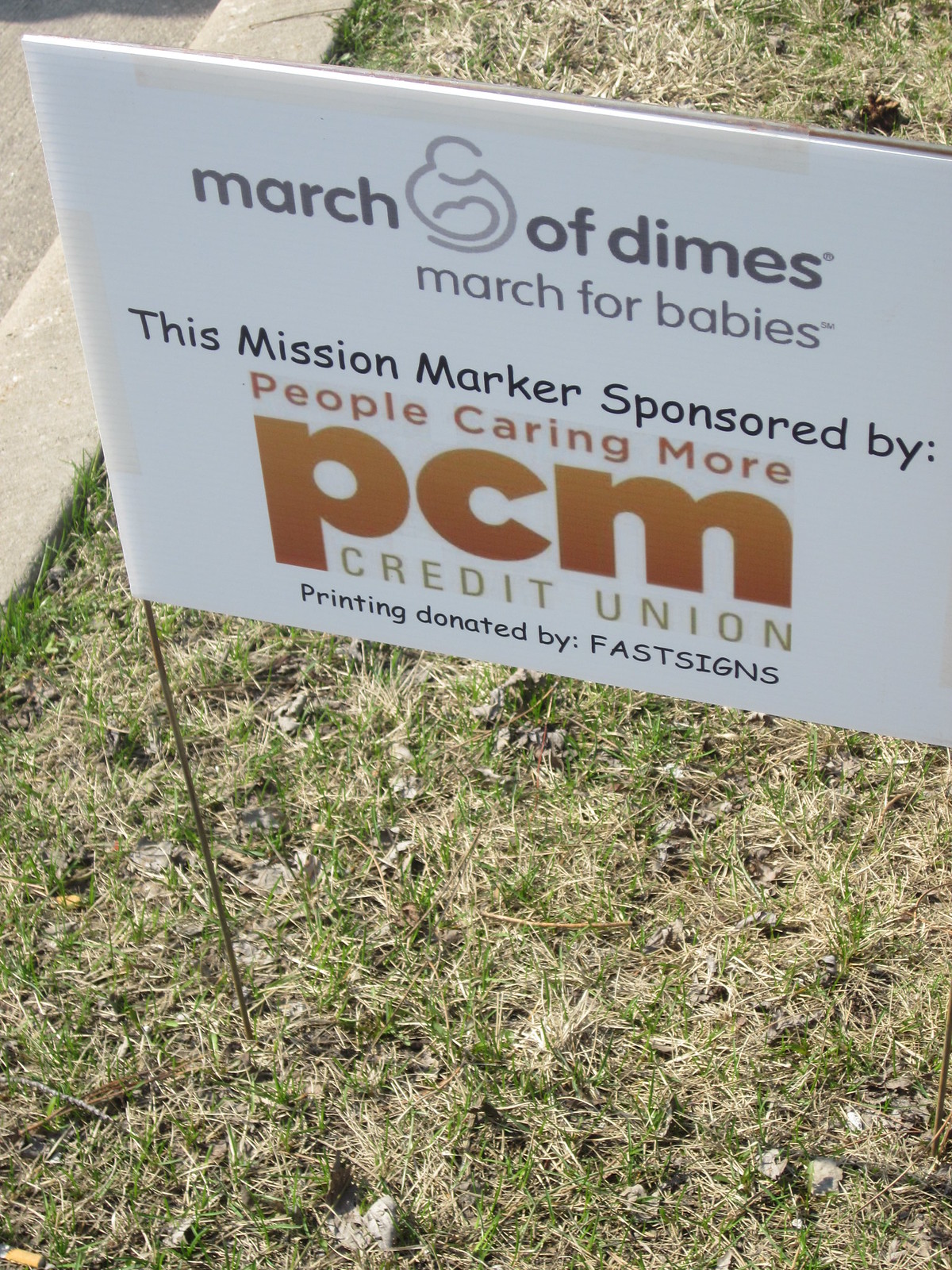This image portrays a white advertisement sign for the March of Dimes, specifically promoting the March for Babies event. The sign is mounted on metal rods and staked into a grassy area that appears green and brown. The grass is contained within a curb, possibly part of a median. The background reveals cement, indicating proximity to a street or sidewalk.

The text on the sign is detailed and informative. At the top, "March of Dimes" is displayed in black print, accompanied by the organization's logo. Below that, the phrase "March for Babies" is printed. The sign further reads, "This mission marker sponsored by People Caring More," with "People Caring More" in smaller, light brown print. Prominently, "PCM Credit Union" is indicated in larger, burnt-orange font. Finally, the footer of the sign notes, "Printing donated by Fast Signs" in smaller black print.

This well-placed sign sits within the grassy boundary next to a curb, effectively catching the eye of passersby in a daytime outdoor setting.